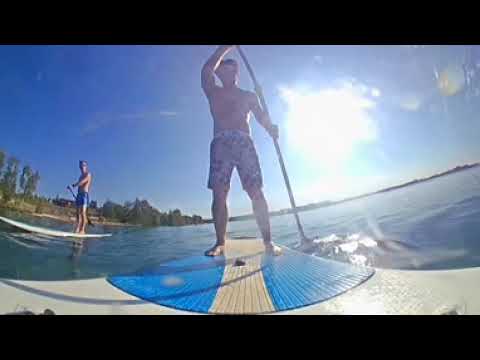On a picturesque summer day, two men are enjoying a paddleboarding adventure on a serene lake. The camera's perspective is mounted low on one of the paddleboards, capturing the scene as if looking up at the closer man. He stands on a white paddleboard with blue sections along the footboard, grasping a long paddle that's submerged in the lake's clear blue water. The man is squinting in the bright sunlight, wearing swim trunks, and appears to be concentrating on navigating. To the left of him, another man stands on a similar white paddleboard, wearing blue swim trunks and holding his paddle ready for the next stroke. The calm water contrasts beautifully with the vibrant green trees lining the distant shoreline. The sky is a perfect blue with the sun glowing brightly in the upper right corner, casting a warm light over the peaceful scene. They seem to be enjoying their youthful energy and the physical activity on this perfect day.